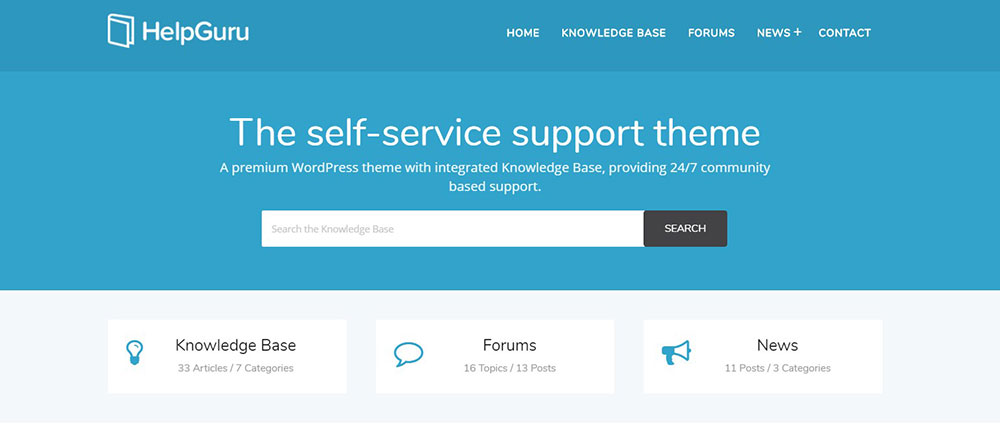In the upper left corner of the image, a book is being opened, symbolizing access to knowledge. To its right, the text "Help Guru" is prominently displayed. Adjacent to this title, a navigation menu lists categories including Home, Knowledge Base, Forums, News, and Contact. Below this menu, in white text against a bright blue background, is the tagline "The Self-Service Support Theme: A premium WordPress theme with integrated knowledge base, providing 24-7 community-based support." Centrally located is a large search bar with the light gray prompt "Search the Knowledge Base," accompanied by a black rectangle with the word "Search" in uppercase letters. Directly below this, the Knowledge Base section features 33 articles across 7 categories. The Forums section, denoted by a speech bubble icon, includes 16 topics and 13 posts. The News section, identified with a megaphone icon, has 11 posts within 3 categories. The background color tying the entire design together is a striking bright blue.